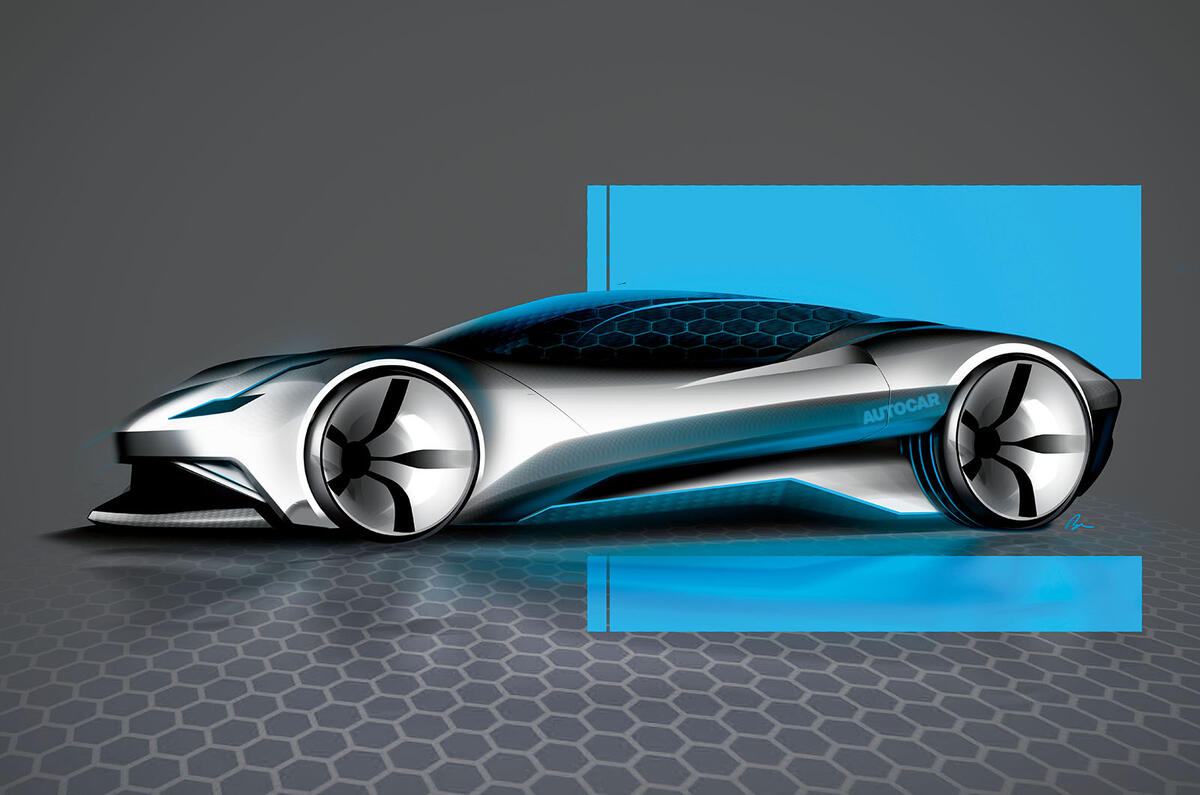In this image, we see a highly detailed, futuristic concept car, set against a light to dark gray gradient background with a honeycomb pattern that fades towards the center. The car, which is silver with blue reflective highlights, occupies the foreground and is positioned horizontally, facing left. Its sleek, smooth body features a flat, roundish front grille with an extended lower lip in black and silver trim. The car boasts an all-glass, blue-tinted roof that seamlessly merges with the curving side windows into a streamlined trunk.

Notable design elements include incredibly thin, black tires adorned with prominent silver rims, and spiral-like wheels that evoke a sense of motion or a journey through a portal. The car's side windows, also made of glass, have a distinctive honeycomb pattern. Enhancing the futuristic appeal, there is a blue square overlay behind the car on the right side, with the words "auto car" near the rear fender rendered in blue. The design is clearly a 3D render or prototype, emphasizing bold, avant-garde automotive aesthetics.